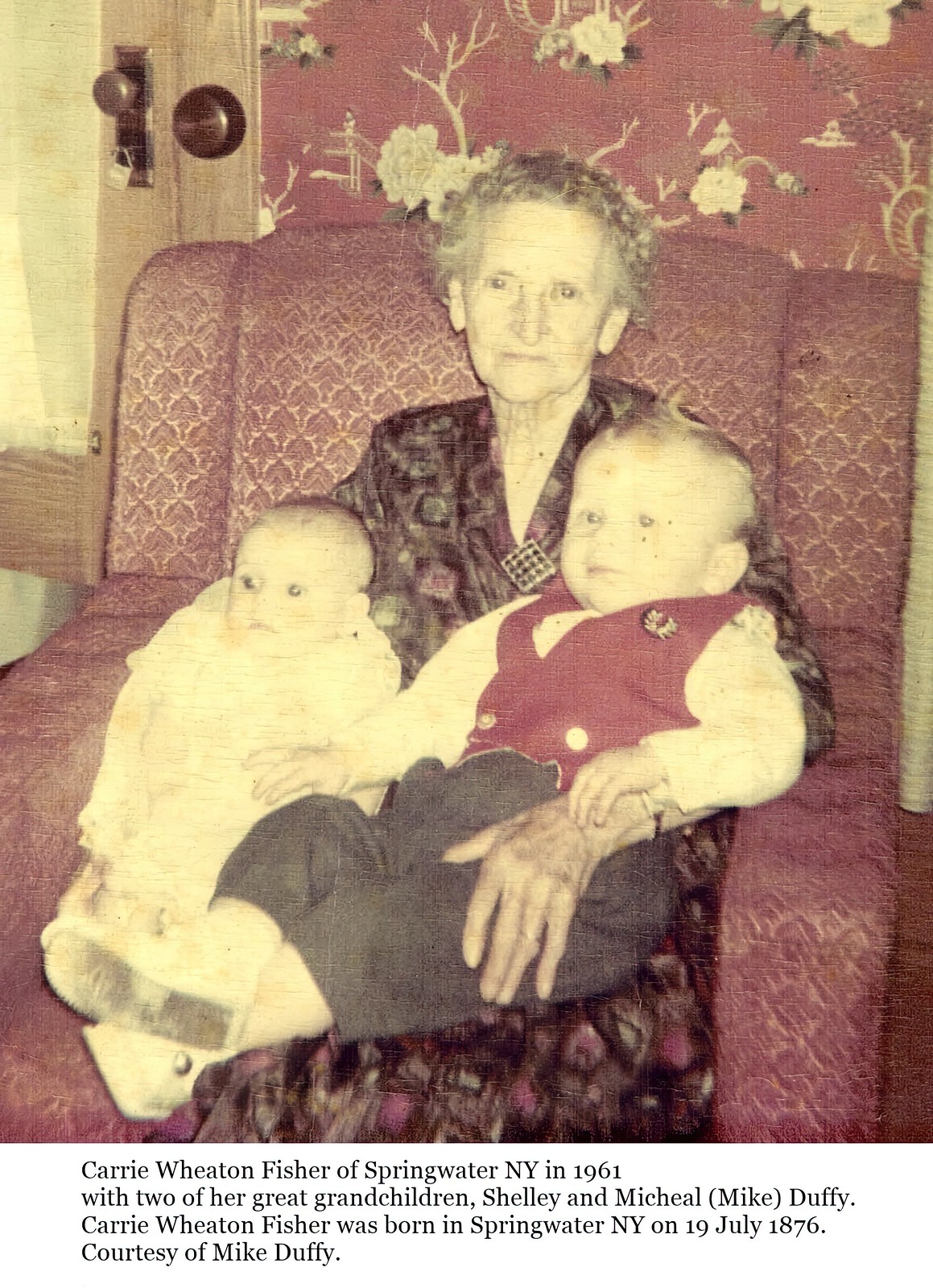In this faded and color-washed photograph from 1961, an elderly Carrie Wheaton Fisher of Springwater, New York, born on July 19, 1876, is seated on a rose-colored couch. She is wearing a purple and black dress adorned with a square, diagonally oriented medallion at her neckline. With her right arm, she cradles a baby dressed in a white garment, nestled comfortably against the couch. In her left arm, she supports a toddler, who sports a reddish vest, blue pants, and whitish shoes. The background features ornate wallpaper with floral and branch designs and a visible door on the upper left side. Beneath the image, a caption reads: "Carrie Wheaton Fisher of Springwater, New York in 1961 with two of her great-grandchildren, Shelly and Michael Mike Duffy." This photograph is courtesy of Mike Duffy.